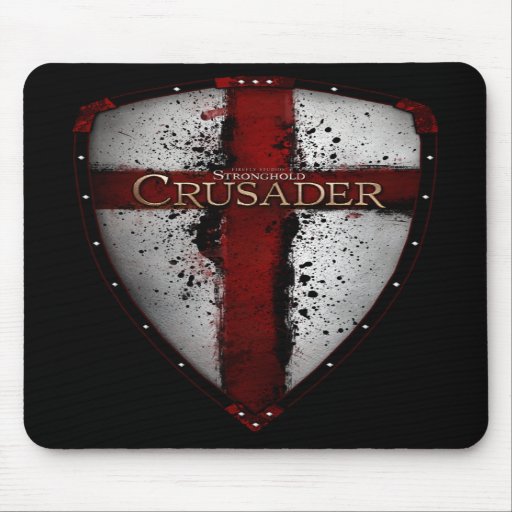The image displays a perfectly aligned mousepad against an eggshell background. The mousepad, roughly four inches square with rounded edges, has a black background. Dominating the center of the mousepad is a shield design with black and white accents. The shield is light gray and features a red cross comprised of two red stripes, with black ink splatters adorning the vertical stripe. The shield is bordered by a dark reddish-black outline detailed with small white dots, simulating bolt placements. In the center of the red cross, in gold lettering, are the words "Firefly Studios," with "Stronghold Crusader" beneath it in gold capital letters. The setup suggests either a product display or a personal showcase.